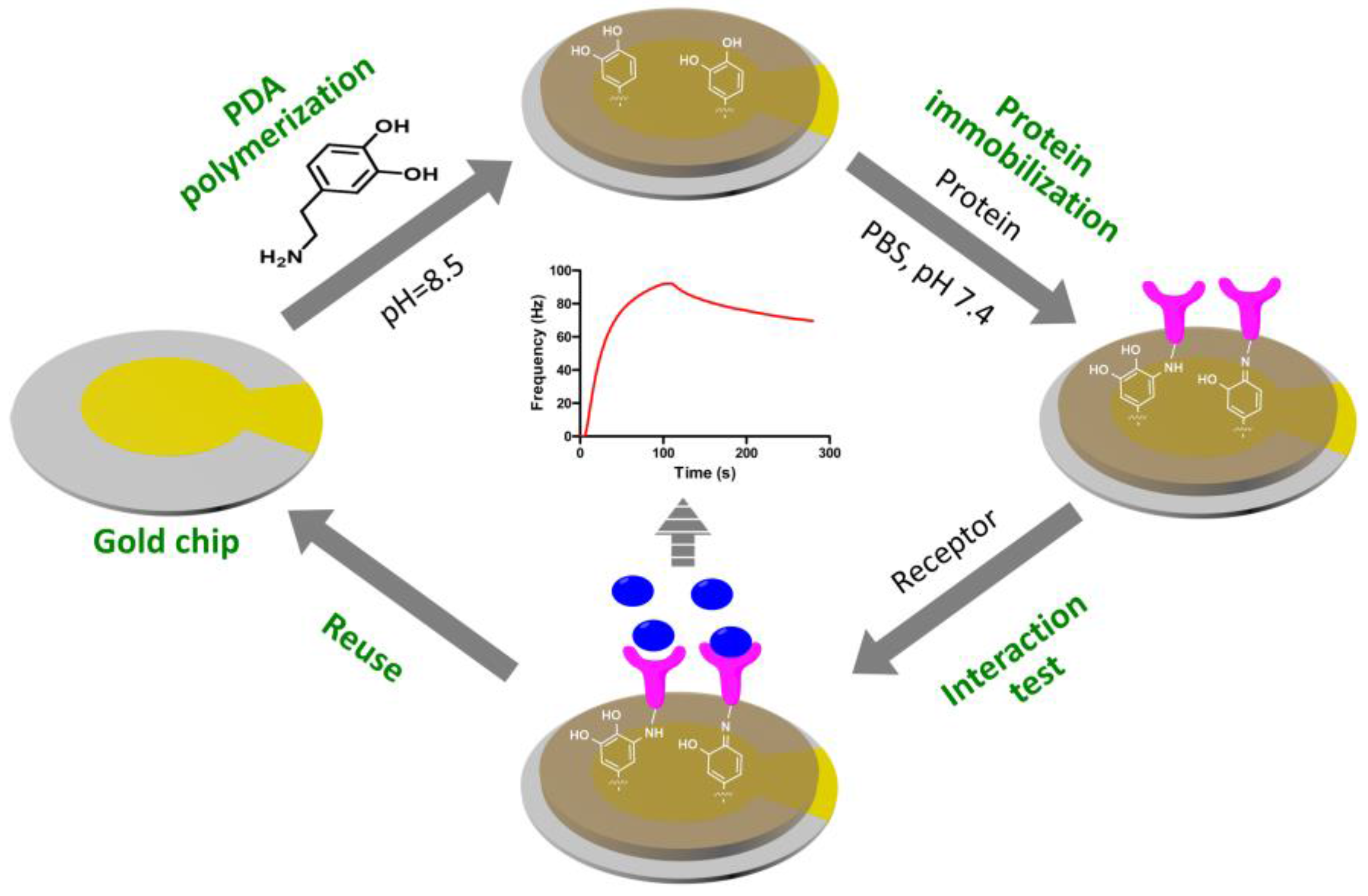This illustration, seemingly from a chemistry textbook, is a detailed depiction of the PDA polymerization process and subsequent protein interactions, represented in a cyclical sequence involving four stages. Arranged in a diamond-shaped layout, the diagram incorporates arrows pointing in a clockwise direction, illustrating the step-by-step progression of the reactions.

1. **Bottom Circle (Gold Chip)**: The starting point shows a gray circle with a central gold disc, labeled "Gold Chip." The illustration indicates gold extending outward from the center, highlighting the chip's active surface.

2. **Left Arrow (PDA Polymerization)**: Moving clockwise to the top circle, an arrow labeled "PDA Polymerization" leads to this stage. Here, the depicted chemical structure shows "H2N" connected to a hexagon with "OH" groups, indicating the polymerization process at a pH of 8.5.

3. **Top Circle (Protein Immobilization)**: The next arrow directs to the right, indicating "Protein Immobilization." This stage shows the modified polymer structure adhering to the gold surface, with the text noting "PBS, pH 7.4." The image specifies the successful attachment of protein molecules, depicted as magenta stick figures with a U-shaped top.

4. **Right Arrow (Receptor Interaction Test)**: Continuing clockwise, the next stage involves the "Receptor Interaction Test." Here, pink structures on the polymer surface interact with blue circular molecules, representing receptor interactions verifying the successful immobilization.

5. **Bottom Arrow (Reuse)**: The final stage labeled "Reuse" loops back to the beginning, signifying the potential reusability of the functionalized gold chip.

**Central Graph**: The middle of the illustration features a graph charting the reaction kinetics, with time (0-300 seconds) on the x-axis and frequency (Hz) on the y-axis. The red line on the graph indicates the frequency changes, peaking shortly after 100 seconds before gradually declining, illustrating the reaction's progress as monitored via the frequency changes.

Overall, this image comprehensively describes the entire process from PDA polymerization to protein immobilization, subsequent receptor interaction, and potential reuse of the gold chip, providing a clear and detailed view of the reactions involved.